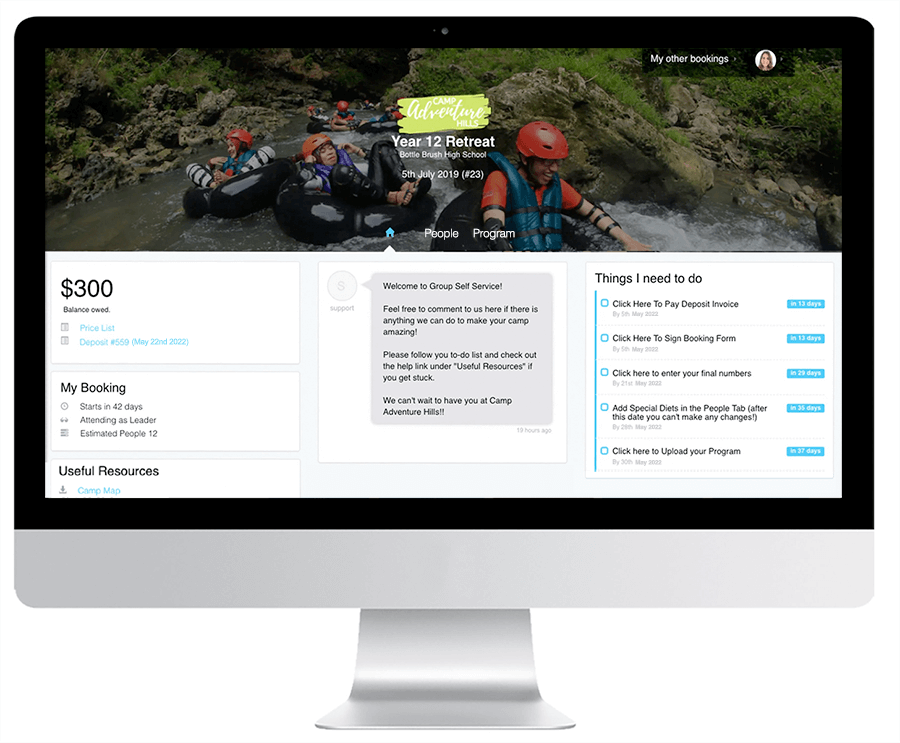Category: Websites

A prominent iMac screen displays a webpage titled "My Other Bookings." The featured booking, "Camp Adventure Hills, Year 12 Retreat, Battle Brush High School," is scheduled for July 5, 2019, with booking number 23. The screen shows an engaging image of six individuals tubing over rapids, each donned in helmets and life vests, surrounded by rocks and lush greenery, capturing the adventure's essence. Below the image, details indicate a $300 balance is still owed, with the booking set to commence in 42 days. The individual is attending as a leader, with an estimated group size of 12. The page also includes a list of useful resources and tasks to complete.